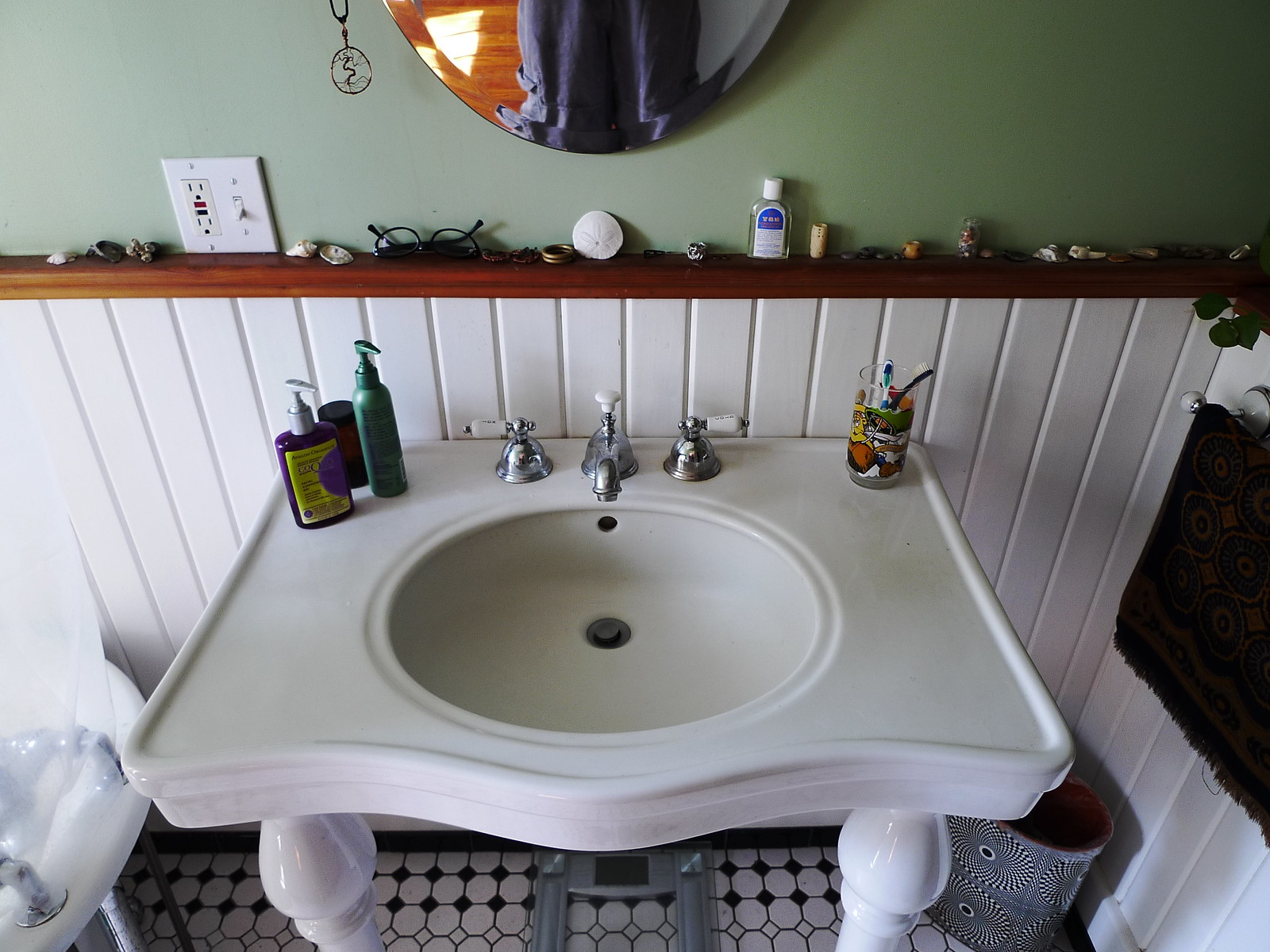A detailed, straight-on view of a bathroom sink reveals a quaint and cozy setting. The walls are painted a soothing sage green, providing a calming backdrop. Above the sink hangs an oval-shaped mirror, reflecting a draped, blue fabric—possibly part of someone's attire—although only the middle portion is visible. Below the mirror, a brown wooden ledge holds various items: a pair of glasses, a collection of seashells, and a bottle of hand sanitizer. To the side, a light switch and an electrical outlet are mounted on the wall.

The lower half of the wall features narrow vertical planks reminiscent of beadboard, painted white. The white ceramic sink itself doesn't have a straight edge; instead, it dips inward to form a gentle curve. Nearby, a cup holds toothbrushes and a bottle of soap. 

In the reflection, an elegant, old-fashioned bathtub is partly visible, adorned with a white overlay. Directly to the right, a black and white garbage can sits on the floor. The flooring is a striking checkered pattern of black and white tiles, completing the vintage-inspired aesthetic of the bathroom.